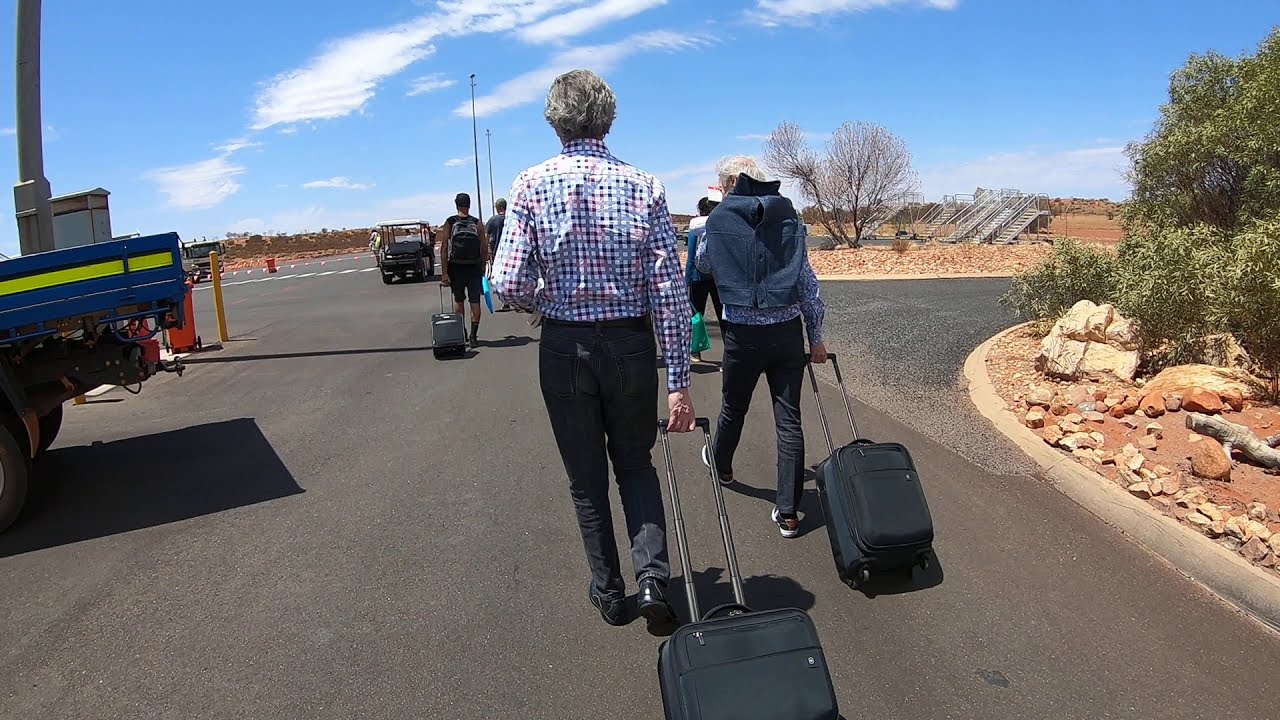In a bustling outdoor scene, likely at an airport parking lot on a bright afternoon, travelers are seen from behind, walking towards their destination. Central to the image are two individuals pulling black roller suitcases with silver handles. The one on the left, an older man with gray hair, dons a multi-colored plaid shirt (featuring red, blue, black, and white), black jeans, and black shoes. Adjacent to him, another person appears to be wearing a jean jacket tied backwards around their neck, a colorful patterned shirt, and dark jeans. Together, they lead the way, with additional travelers in the background also toting their luggage. To the far left, a parked truck and a pole are notable, alongside light poles that recede into the distance. The sky is predominantly blue with fair weather cumulus clouds, and hints of a wide road and curbs with brown soil and rock formations, as well as some sparse greenery and desert-like rocks. Distant ramps hint at the airport's proximity, completing a vivid snapshot of a travel day.